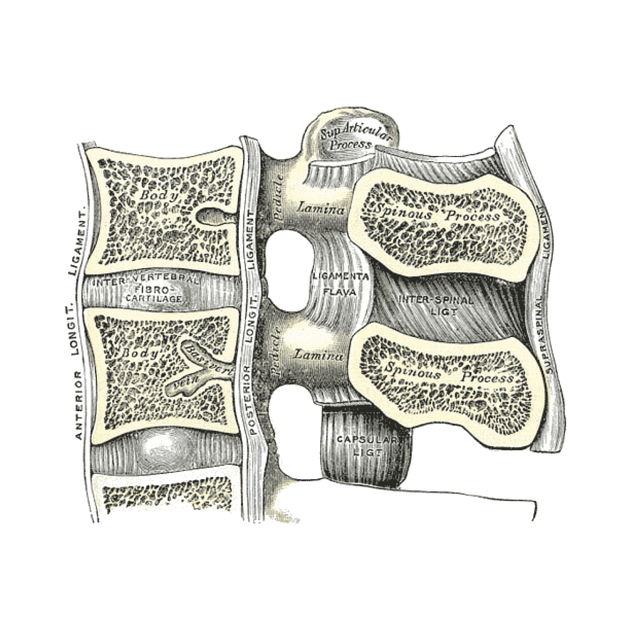This intricately detailed, hand-drawn anatomical diagram depicts a longitudinal cross-section of the spine against a white background. The left portion of the image features labeled components including 'anterior longitudinal ligament,' 'posterior longitudinal ligament,' and 'intervertebral fibrocartilage,' alongside three stacked vertebrae. The spine's cutaway view reveals square-shaped vertebral bodies labeled 'body,' interconnected by intervertebral fibrocartilage. To the right, the diagram highlights elements such as the 'spinous process,' 'spinous process ligament,' 'supraspinal ligament,' and 'interspinous ligament.' The middle of the image showcases central spinal components with labels like 'superior articular process,' 'lamina,' 'pedicle,' 'ligamenta flava,' and 'capsular ligament.' The overall drawing, sketched in shades of black and white with a hint of yellowish beige, provides a comprehensive view of the spine's anatomical structure, including various ligaments and cartilaginous elements.